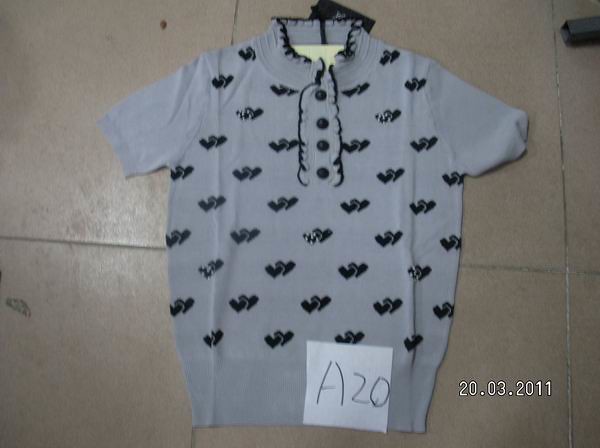A white t-shirt with a high neckline prominently featuring black stitching is hanging on a hanger against a pale beige wall. The shirt is adorned with an all-over pattern of black and grey heart pairs. Four black buttons run down the front from the collar to the chest area. The waistband of the shirt is distinctively knitted and ribbed, providing a stretchy fit. Toward the bottom of the image, a white notice is visible, displaying the text "A20" alongside a date, "20th of March, 2011."